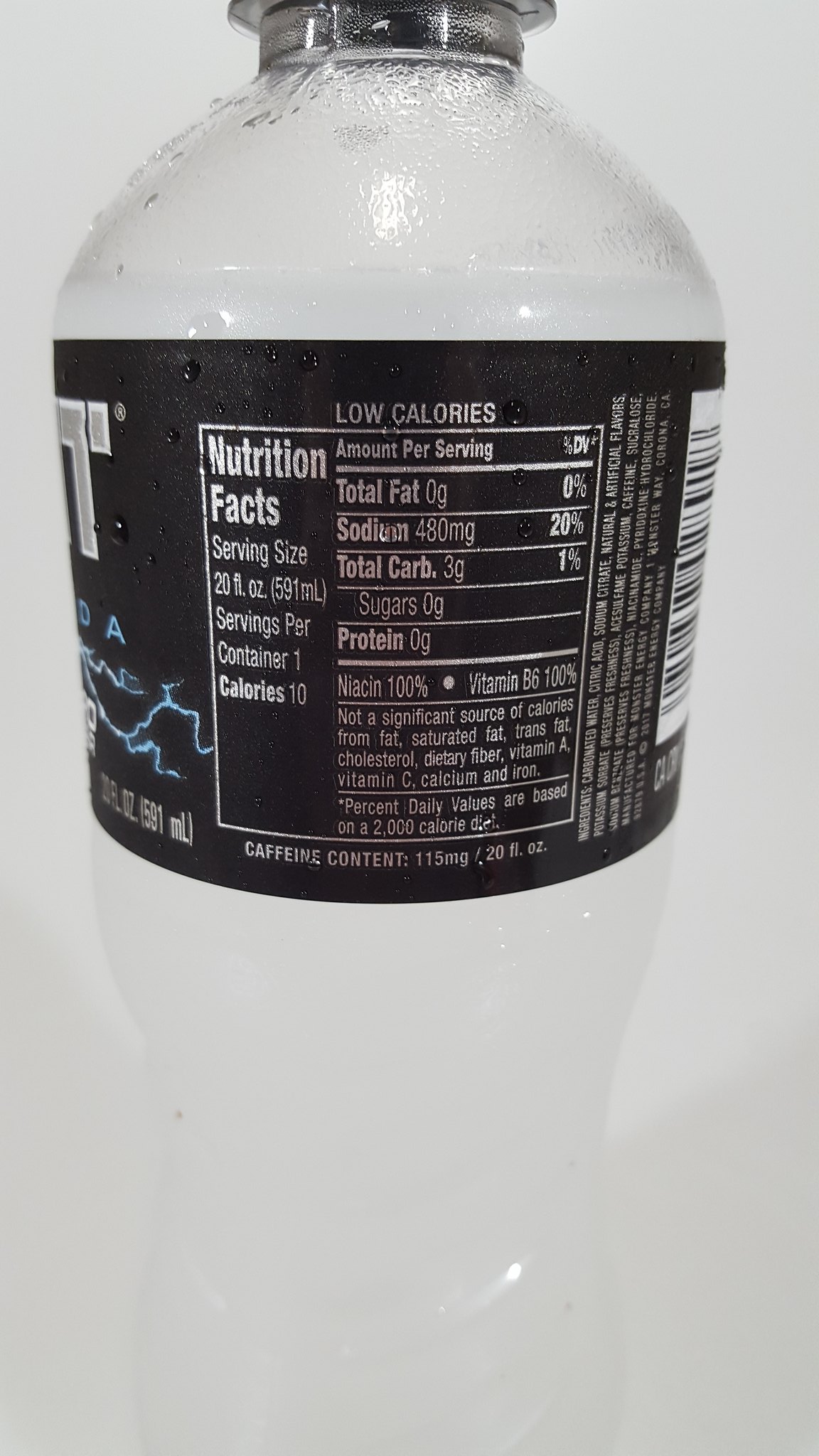The photograph features a clear bottle of an energy drink with a cloudy liquid inside, resembling murky water. The bottle has a black label adorned with silver, blue, and white text. Prominently displayed on the label are blue lightning strikes. The visible portion of the brand name ends in the letter 'T' while another part shows 'DA'. The nutritional information is detailed, highlighting the drink's low calorie content and absence of fat, sugars, and proteins. For a serving size of 20 fluid ounces, it provides 110 calories, 0 grams of fat, 400 milligrams of sodium (20% daily value), 3 grams of total carbohydrates (1% daily value), 0 grams of sugars, and 0 grams of proteins. The drink also contains 100% of the daily recommended intake of niacin and vitamin B6, along with 115 milligrams of caffeine per 20 fluid ounces. The label specifies that it is not a significant source of calories from fat, saturated fat, trans fat, cholesterol, dietary fiber, vitamin A, vitamin C, calcium, and iron. The barcode is partially visible in the photograph, suggesting it might be an image intended for online display to inform buyers about the product's nutritional content.